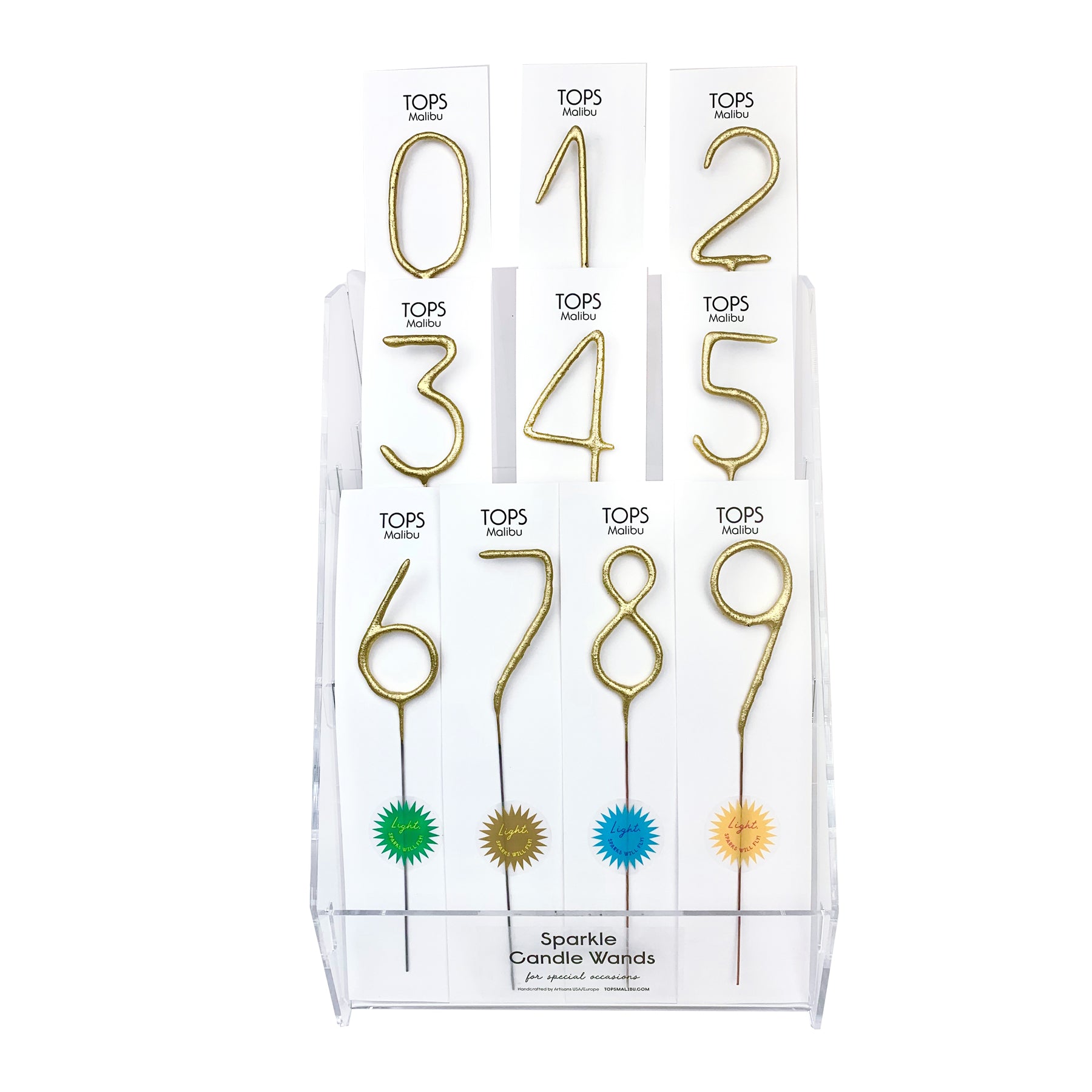This photograph captures a display stand showcasing Sparkle Candle Wands by TOPS Malibu. The display holder, which is translucent, features three rows of candle wands, each displaying a gold-colored number from 0 to 9. The numbers are arranged sequentially: 0 through 2 on the top row, 3 through 5 in the middle, and 6 through 9 on the bottom row. Each number is mounted on an individual piece of white cardboard with a black label at the top reading "TOPS MALIBU," where "TOPS" is prominently larger and in all caps. These wands appear to be designed for special occasions, such as birthdays, and each comes with a thin rod attachment, resembling a needle, for easy placement on cakes. Underneath the numbers, various colored sparkles—green, brown, blue, and gold—add a festive touch. The bottom section of the display is labeled "Sparkle Candle Wands," followed by a scripted note, "for special occasions." The overall image has a clean, white background, highlighting the product's elegant design and purpose.